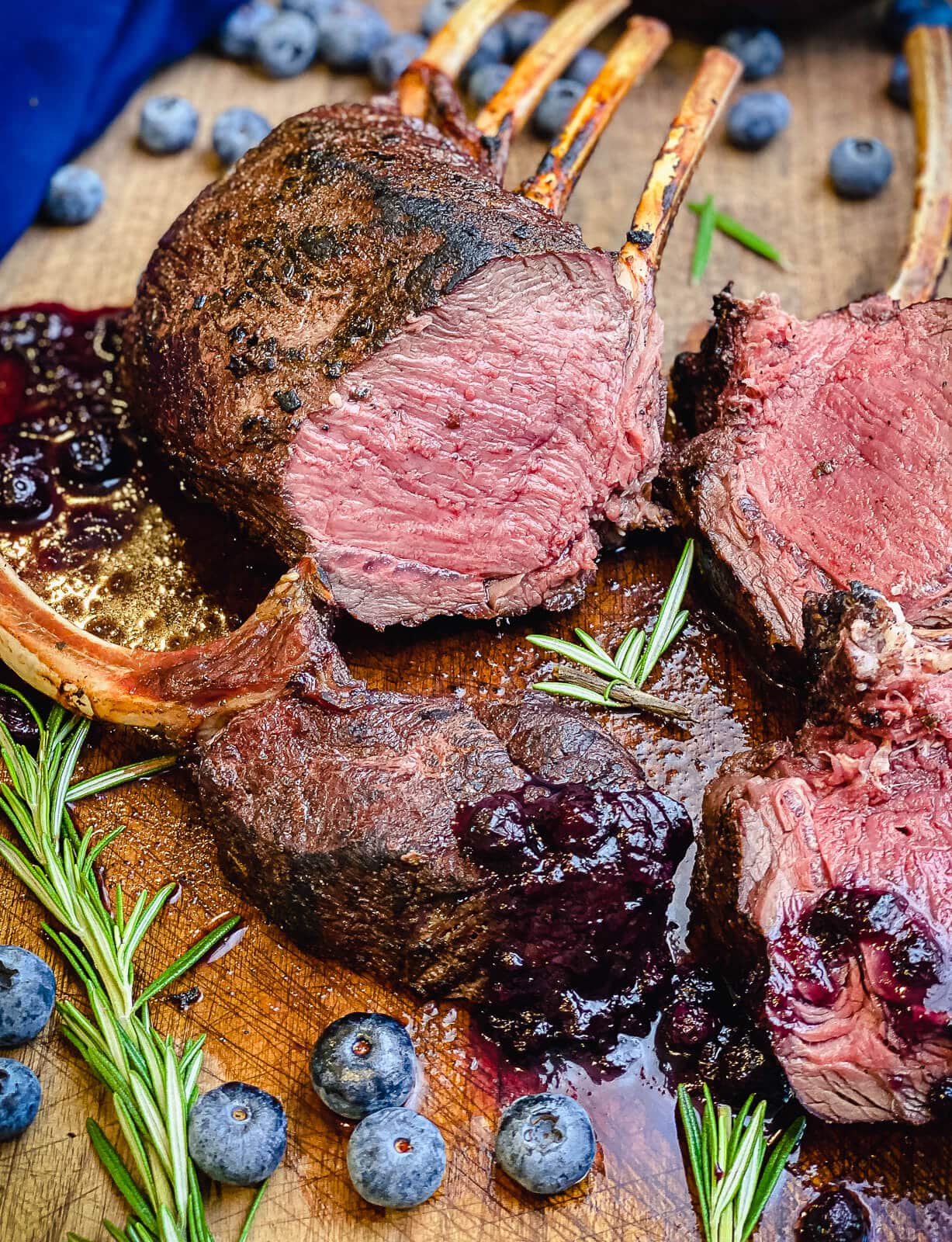This image showcases a beautifully presented brisket on a rustic wooden cutting board. The brisket features a charred, brown exterior that contrasts vividly with its juicy, pinkish interior. Some bones are still embedded within the meat, while others are set to the side. A dark, purplish sauce, likely cranberry, adds a glossy sheen to portions of the brisket and spills onto the cutting board. Scattered around the brisket are sprigs of rosemary and numerous blueberries, both on the cutting board and blurred in the background, adding a fresh touch to the scene. The upper left corner of the image includes a hint of a blue fabric, complementing the overall composition.